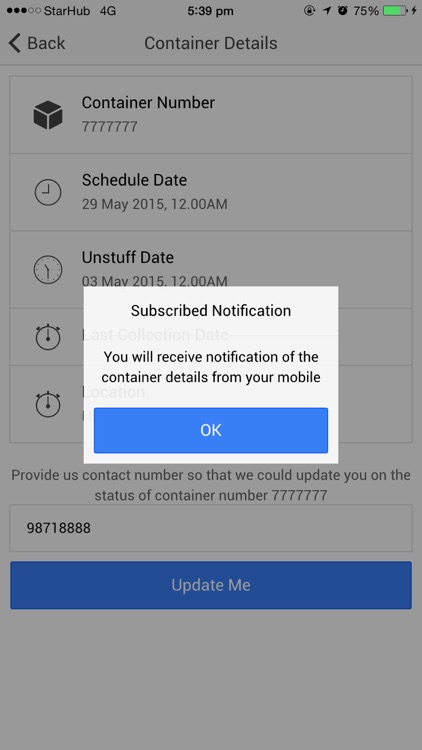A screenshot of a mobile phone screen displays various UI elements related to container tracking details. 

In the top-left corner of the screen, the signal strength is indicated by five dots, three of which are filled in black, next to the text "StarHub 4G." The top-center shows the current time, "5:39 PM," and on the top-right, there is a battery icon filled to 75% in green, accompanied by the number "75%" and a small clock icon.

Just below this top bar, the screen shows a title that reads "Container Details" against a gray-shaded background. To the left of this title is a "Back" button with an arrow pointing to the left. A thin gray line divides this section from the detailed information below.

The first line of details lists "Container Number" in black text next to a black 3D box icon displaying three visible sides. Below this, the container number "777-7777" is prominently displayed. Following another thin gray line, the second detail is labeled "Schedule Date" in black with a clock icon outlined in gray, showing "29 May 2015, 12 AM."

Another gray line separates this from the third detail, "Unstuffed Date," also accompanied by a gray-outlined clock icon, which states "03 May 2015, 12 AM."

Partially overlaying the screen is a white notification banner with the message, "Subscribe Notification. You will receive notification of the container details from your mobile," in black text. Below this, a blue "OK" button is visible, which can be tapped to dismiss the notification.

Behind the notification, two more timestamped details can be seen but are obscured. Beneath the banner, a message reads, "Provide Us Contact Number so we could update you on the status of container number 777-7777."

Following this, there is a large gray-outlined box containing the contact number "987-18888" in black. At the bottom of the screen, another large blue banner features the prompt "Update Me" in white text. The screen's lower section returns to a gray background.